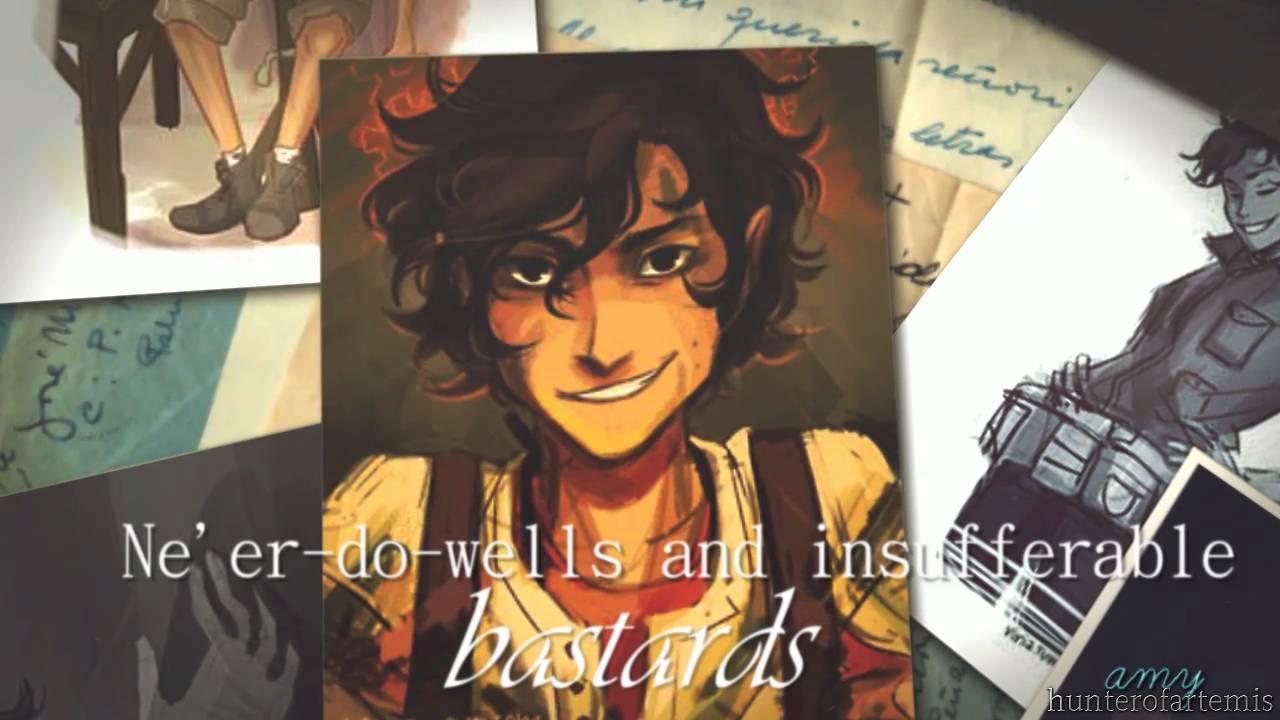The image is a compilation of an artist's diverse works, each distinct in its own context but collectively forming a rich tapestry of creativity. In the top-left corner, an intricate drawing depicts the lower half of a Caucasian person sitting on a chair. The individual is wearing white socks and boots, positioned next to table legs. Directly beneath this drawing, a piece of blue paper with blue text is visible, although its content appears insignificant. Below this, the composition includes a section with a black background adorned by a minimalist white hand drawing. 

To the far right, there is a detailed portrait of a man with wavy brown hair, smiling warmly. He is dressed in a coat and a belt, and appears to be wearing regular pants. 

The centerpiece of the image captures significant attention: it is a larger portrayal of the same man, likely, with curly brown hair and a friendly expression. He appears Caucasian and is dressed in a white shirt with noticeable straps on both sides, layered over an undershirt. 

On the bottom right corner of the image, a watermark reads "Hunter of Artemis," while above this, the name "Amy" is inscribed in blue. Overlaying the entirety of the image is white text proclaiming "Ne'er-do-wells and Insufferable Bastards," adding a final thematic touch to the collection.